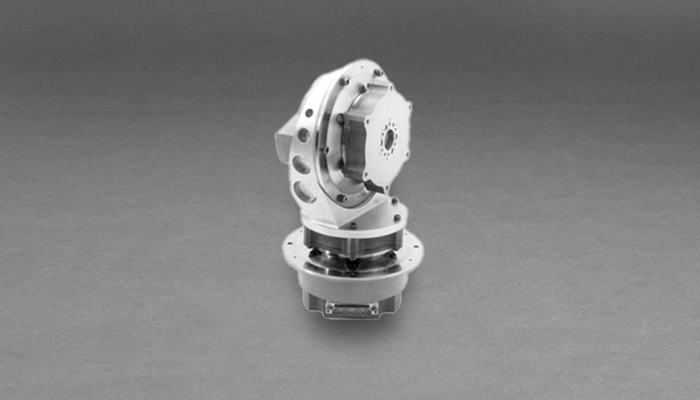Centered in the image is a highly detailed, chrome metallic device, possibly electronic or mechanical in nature. The apparatus features a prominent circular base with a vertically oriented circular component perched atop, seemingly mounted on a swivel that allows for rotational movement. Distinctly visible are the six nodes on the gear-like structure integrated into the upper circular part, which has several holes near its edges, as well as one central hole. The entire object is set against a grey background with a mottled gradient, darkening from the top to bottom, giving it a floating, context-less appearance. The photograph, taken from a side angle, emphasizes the object's intricate design and its varied metallic hues of silver and grey, suggesting an intentional focus on the mechanism itself in an isolated, possibly studio setting.